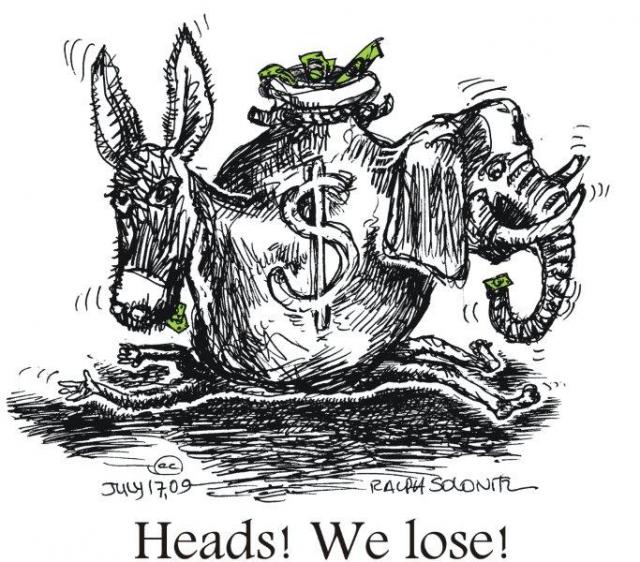The image is a detailed, cartoonish political satire illustration with a white background. Central to the image is a money bag adorned with a prominent dollar sign. Emerging from the money bag are the heads of a donkey and an elephant, representing the Democratic and Republican parties. The creatures are poised on either side of the money bag, greedily consuming green dollar bills, indicative of political greed. The money bag appears to have collapsed onto an unseen person, as evidenced by their arms and legs protruding from beneath it. Handwritten text on the bottom left of the image reads "July 17th, 09" and on the right appears to be signed "Ralph, so on till." Bold, typewriter-style text at the bottom center declares, "Heads! We lose!" The color palette includes black, white, gray, and green, further emphasizing the financial theme. The overall style and composition suggest it is a meticulously crafted political cartoon.